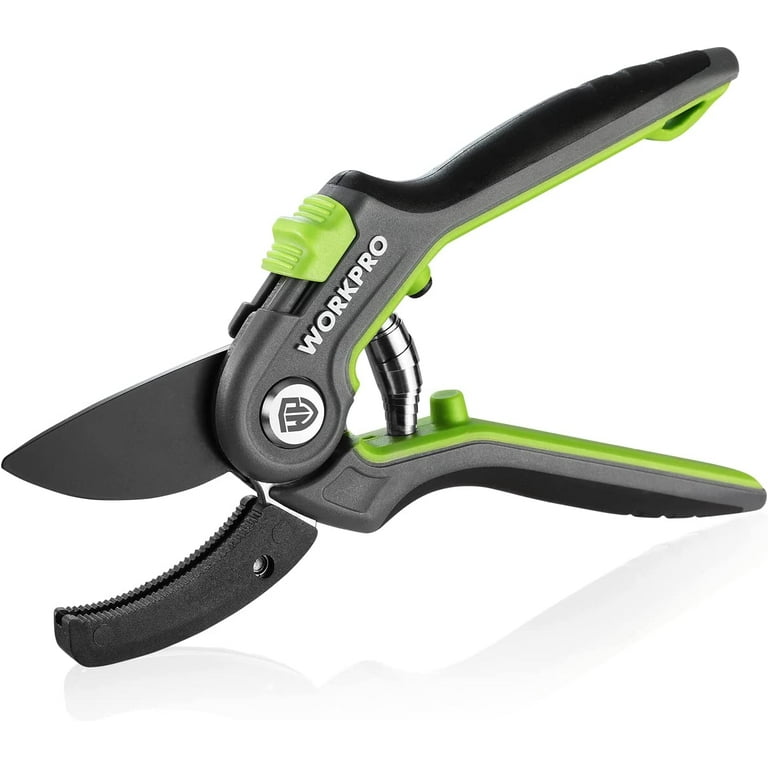This is a close-up image of a tool branded as WorkPro, placed against a plain white background, suggesting it is intended for a sales listing. The tool is primarily made of black and lime green materials. It appears to be a type of adjustable gardening shears or clippers, likely used for cutting tree branches, leaves, or similar outdoor tasks. The tool features ergonomic handles spread apart in a wishbone shape, with lime green trim on the inside. The handles include a green sliding safety mechanism designed to lock the shear closed and prevent accidental injuries. There is a small silver circle in the middle with the letters "W" and "P", confirming the WorkPro brand, which is also printed in white letters along the handle. The blade, which is currently open, is black and connects into a black holder when the handles are squeezed. The overall design highlights functional use and brand visibility.